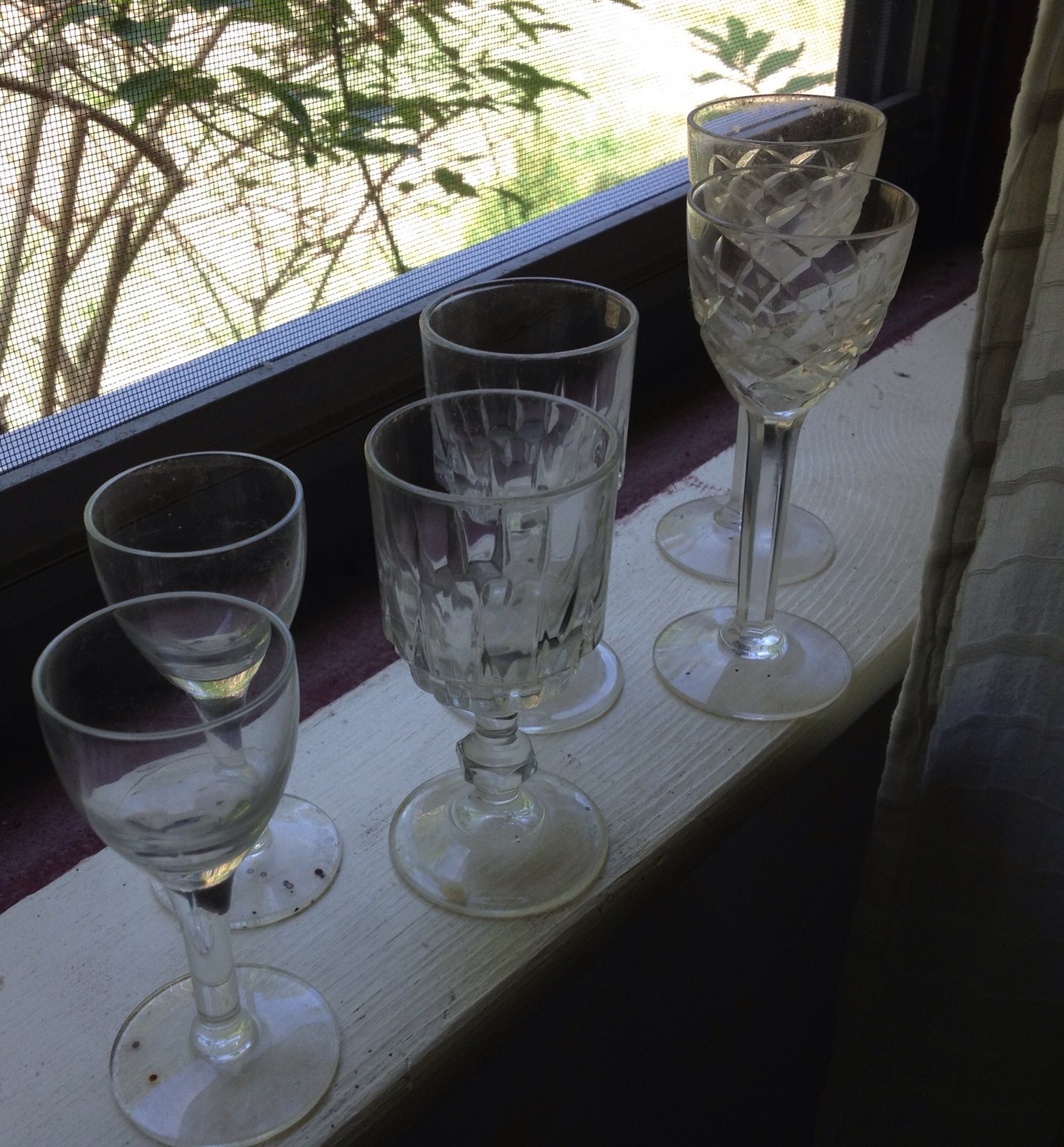This color photograph features six crystal glasses elegantly arranged on a plain, unstained wooden ledge in front of a window. The window, partially covered by a gray curtain, allows a view of a sunlit scene with greenery, including what appears to be bushes or tree branches seen through a mesh screen. The collection includes a variety of shapes and styles: the first glass on the left is a medium-stemmed wine glass, followed by a similar crystal wine glass. The third and fourth glasses are taller, fluted crystal wine glasses with intricate cut designs. Returning towards the center, there is a short-stemmed, traditional drinking glass, commonly used for scotch. Rounding out the display is another crystal wine glass, consistent in style with the first two. Some glasses feature a faceted, cut crystal look, while others have a smooth surface. The arrangement of these glasses against a darker backdrop creates a refined and timeless aesthetic.